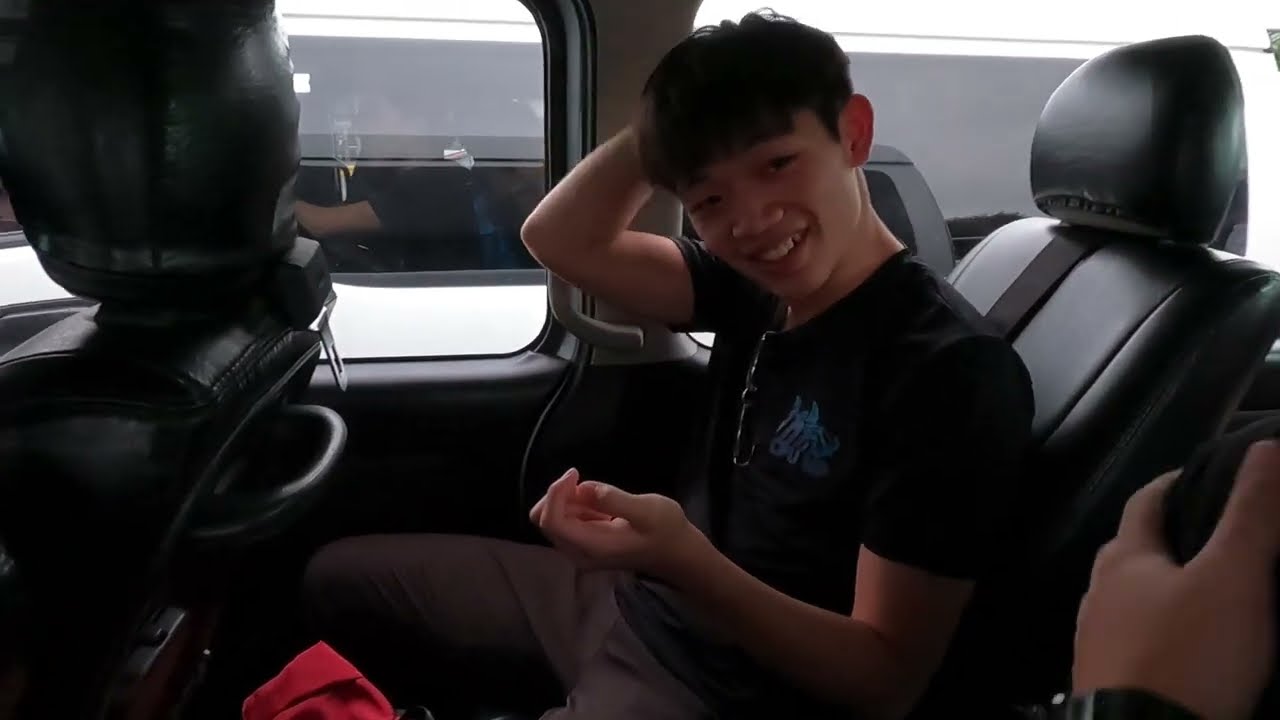The image depicts a young male with short dark brown hair, dressed in a black t-shirt featuring a biking logo over the left breast, paired with light-colored brown pants. He is seated in the backseat of what appears to be a van. His right arm is raised and bent behind his head, as if scratching it, and he is smiling warmly at the camera. Around his neck, a silver chain is visible. The interior of the van is predominantly black and gray, featuring a black chair directly in front of him. Next to him, the right hand of another individual can be seen. Visible through the van’s windows is another vehicle, also a van, with multiple people inside. The bright daylight outside contrasts with the darker tones inside the van, highlighting that the photo was taken during the day.